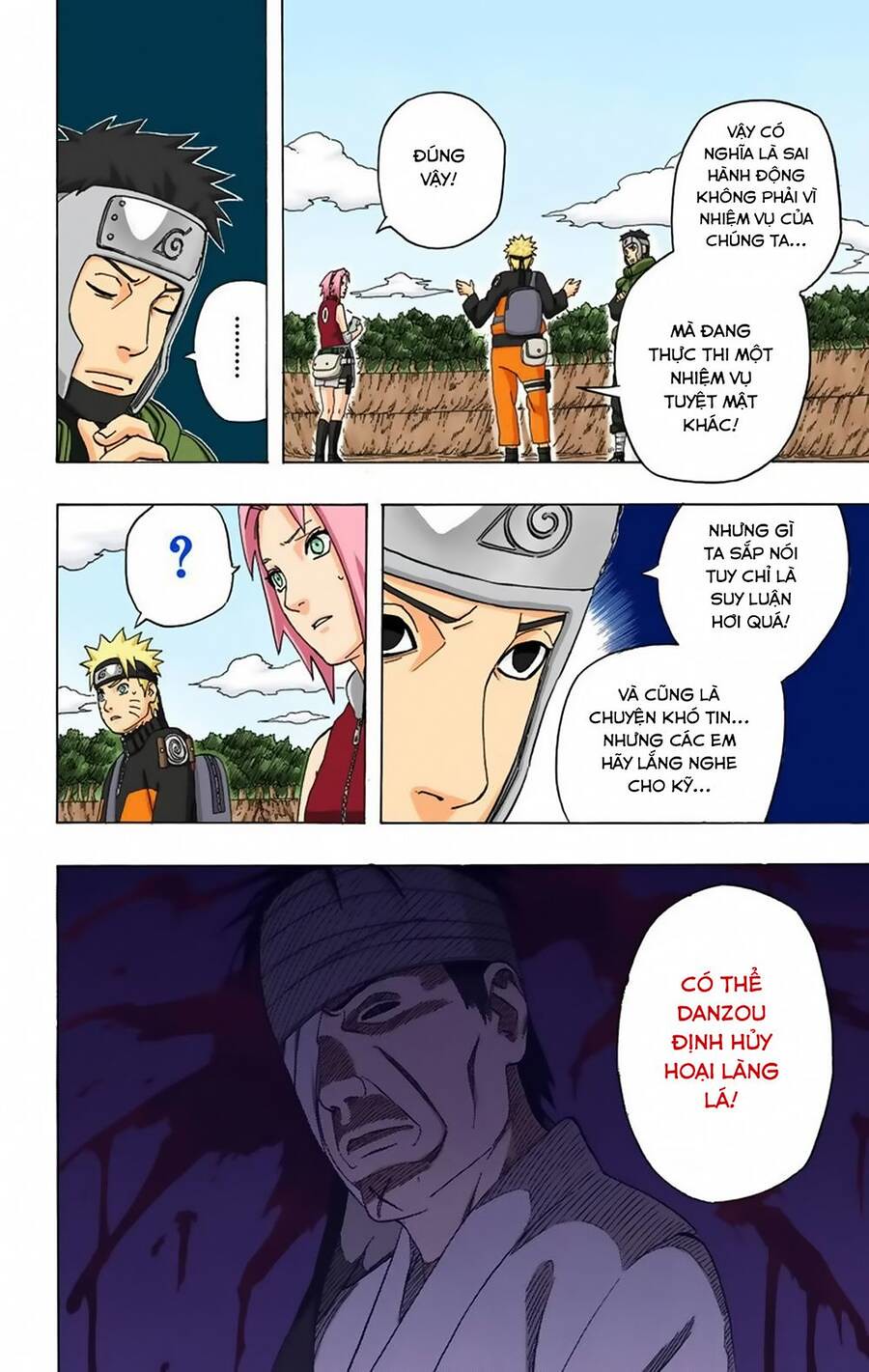The image depicts a richly detailed comic book page segmented into three primary sections. In the top-left vertical frame, a light-skinned man with spiky black hair, a metallic warrior helmet, and shocked expression, murmurs something indistinct represented by ellipses within a speech balloon. To the right, a larger box showcases a sunny scene with a blue sky, fluffy white clouds, trees, and possibly a staircase or brown wall. In this frame, three characters stand together: a woman on the left with pink hair and a red blouse, a central figure with yellow spiky hair, an orange outfit, a purple backpack (resembling a skydiver), and another man to the right. They appear to be speaking in what looks like Vietnamese, with multiple dialogue bubbles appearing around them.

The middle section repeats the backdrop of a blue sky with white clouds, trees, and a brown wall. It zeroes in on the woman with pink hair and the central figure with the yellow spiky hair from the previous frame. Both have question marks in their speech bubbles, indicating confusion or curiosity. Next to this, another frame features the helmeted man again, this time with his eyes open, looking intently to the right with a backdrop of blue and white.

The bottom section presents a dark purple frame showing a gravely injured person with a bandaged head and eyes tightly shut, leaning against a wall. Blood spatters suggest a serious head injury. Red text encircles this figure, possibly indicating urgent, dramatic dialogue in Vietnamese, adding to the intensity of the scene.